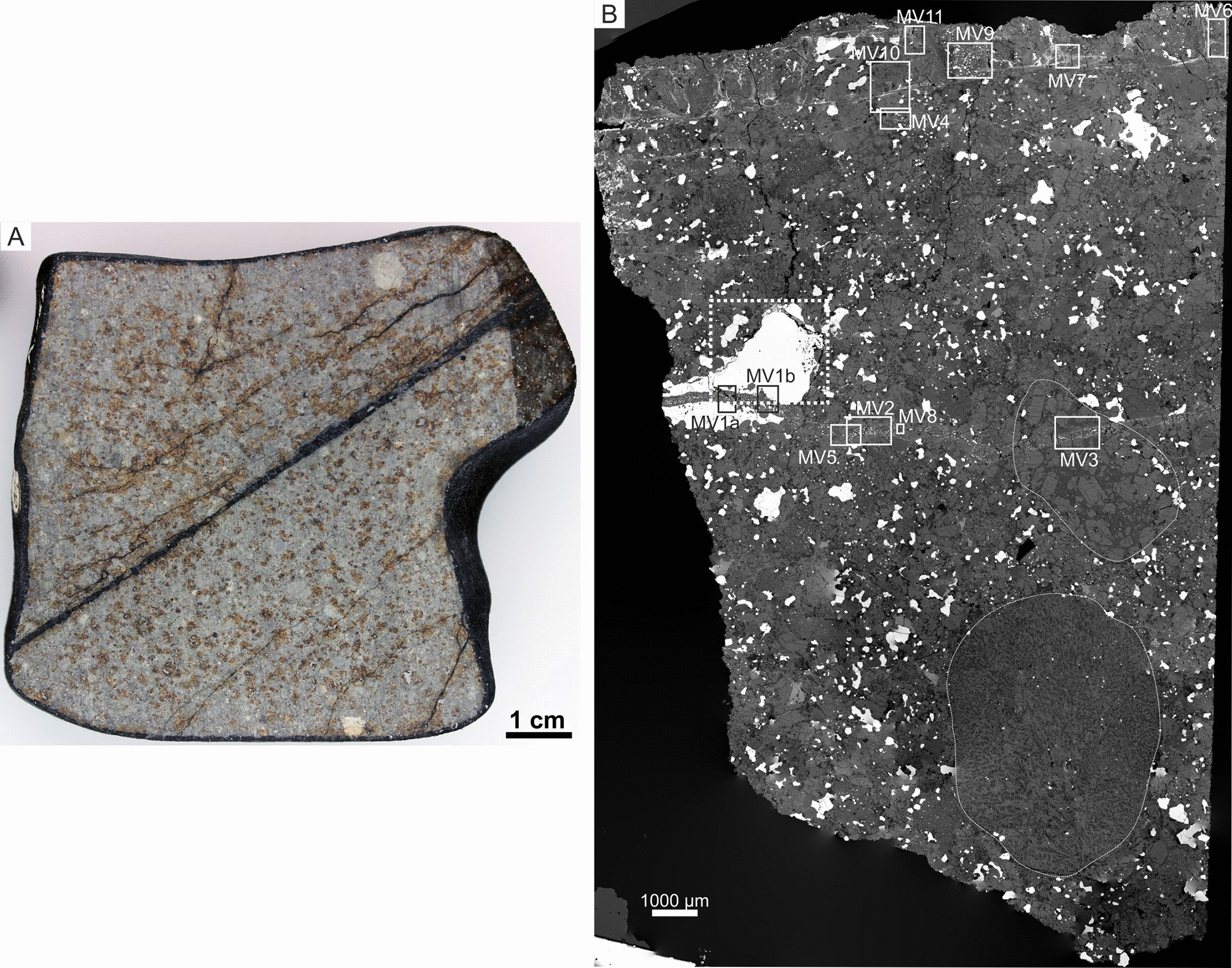The image presents two detailed photographs of a rock, arranged side by side. The left image, labeled "A," shows a somewhat square-shaped rock with a rounded bit near the top right, featuring a prominent crack stretching from the bottom left to the top right. This rock exhibits a variety of textures and colors including gray, tan, black, and white, along with brown spots and numerous smaller cracks. On this image, a scale bar indicates the distance of one centimeter.

The right image, labeled "B," appears to be a highly magnified close-up of the same rock, possibly captured under a microscope, offering intricate details of its surface. This magnified view includes several delineated white boxes with labels such as "MB 1B," "MB 1A," "MB 5," "MB 2," "MB 8," "MB 3," and "MV" up to "11," suggesting the rock is being examined for scientific purposes. A measurement key indicating 1,000 micrometers is also present, reinforcing the microscopic nature of this detailed zoomed-in image.

Together, these images provide a comprehensive examination of the rock, showcasing both its macroscopic appearance and its microscopic structural details.